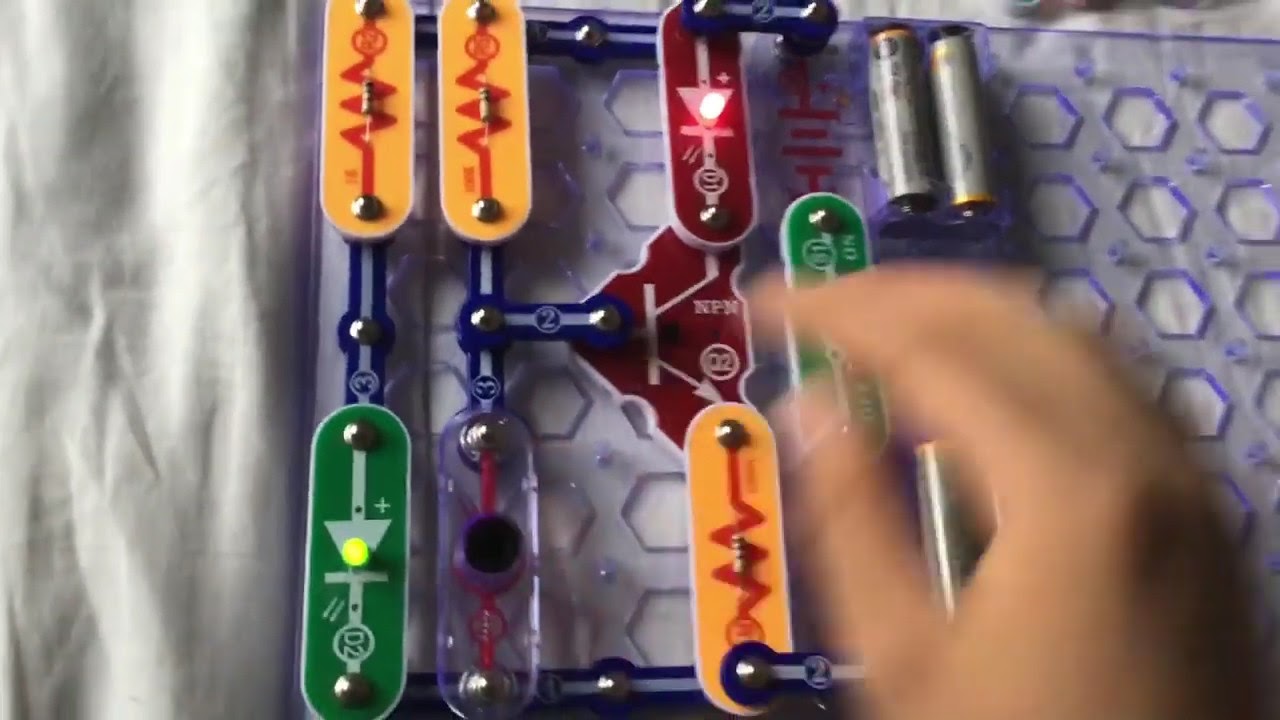The image depicts a detailed view of a scientific or engineering kit focused on teaching electricity and circuits. The setup rests on a wrinkled white cloth, with clear acrylic plastic as the base, featuring hexagon cutouts arranged in rows and columns. Various pill-shaped, oval components, resembling long skateboard shapes, are distributed on the plastic sheet, primarily on the left side. On the upper left, two yellow ovals with red zigzag lines symbolizing electrical current and transistors are visible. In the middle, a green oval with a white arrow and a green LED, alongside a clear oval containing a black component, are prominent. Lower down, another yellow oval with an orange electrical symbol and a transistor is seen, while above it, a red oval with a white arrow points to a red LED. On the right side of the image, there are brackets holding two batteries. The bottom corner of the image shows a blurry hand in motion, seemingly interacting with a red panel featuring a lit-up LED and an arrow, underscoring the dynamic, hands-on nature of the kit.